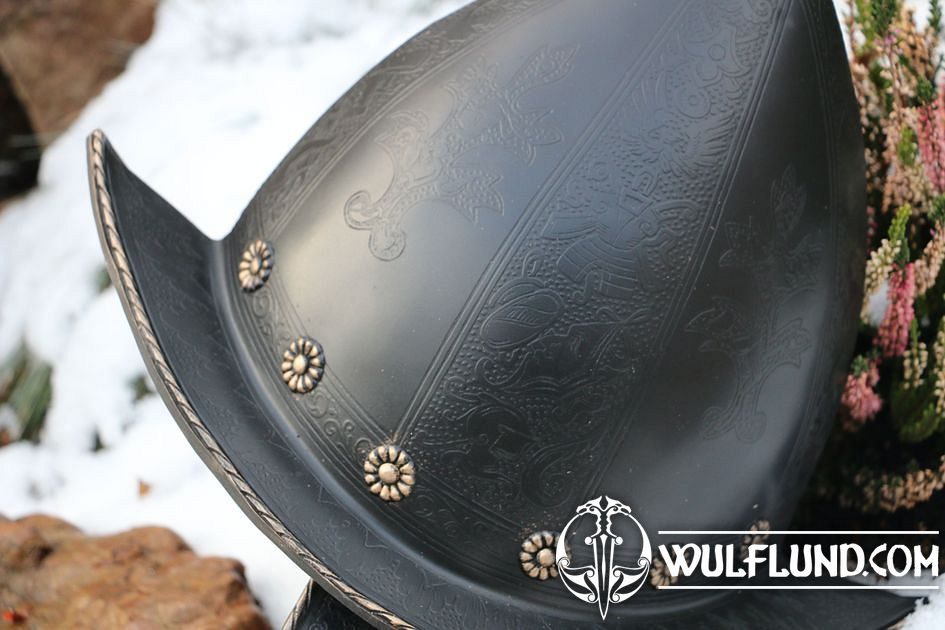This close-up photograph from wolflund.com showcases an ornate black helmet with silver trim and detailed etchings. The intricate floral imprints and three silver flowers embellish the lower part of the helmet, giving it a regal appearance akin to those worn by the Swiss Guards at the Vatican. The textured, metallic surface of the helmet contrasts with the diverse background: on the left, the ground is rocky and snowy, while on the right, pink and white wildflowers thrive among greenery. In the lower right corner, the text "wolflund.com" appears alongside a stylized dagger logo, adding to the helmet's historical and artistic allure.